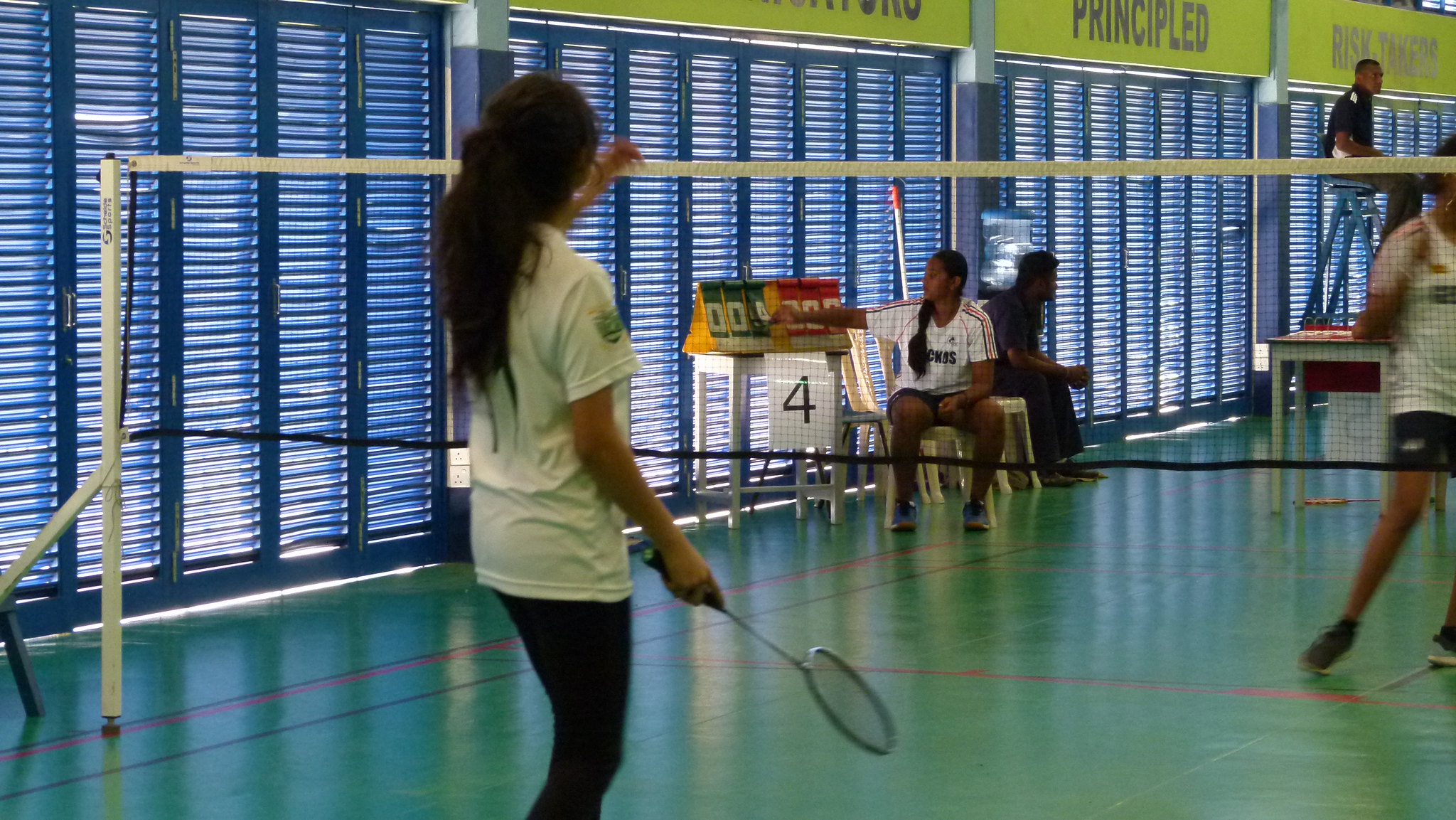The image captures an intense badminton match inside a brightly lit gymnasium with distinct blue and white walls featuring blue shutters. The court's green flooring is marked with red and black lines. In the foreground, a young woman with long brown hair, dressed in a white t-shirt and dark trousers, is poised to serve, holding a racquet in her right hand and lifting her left hand towards the net. Opposite her, another woman in a white t-shirt and black shorts moves to return the serve. The net stretches across the center of the image, anchored by a white pole on the left. Behind the players, two scorekeepers are seated at mid-court, one facing the camera while the other looks away. They sit near a table stand displaying a '4' on a white piece of paper along with red and green markers. In the upper right corner, another judge, dressed in a dark shirt, oversees the match from a raised blue seat positioned along the bluish wall. Yellow signs with blue lettering, including the word "principled," are partially visible in the background, contributing to the organized and official atmosphere of the tournament setting.